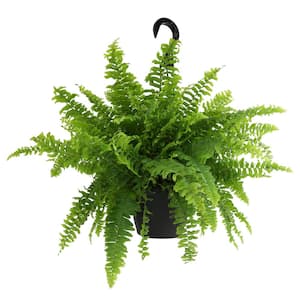The image showcases a vibrant green fern in a six-inch black hanging pot against a white background. The fern is notably full and lush, with fluffy, feather-like leaves extending in all directions, creating a vivid and dynamic display reminiscent of a green firework. The dense foliage nearly conceals much of the pot, emphasizing the plant's abundant growth. At the top, a black plastic hook is visible, indicating that the plant is designed to be hung. The minimalistic backdrop allows the fern's bright, vibrant green color to stand out prominently, highlighting its decorative appeal.